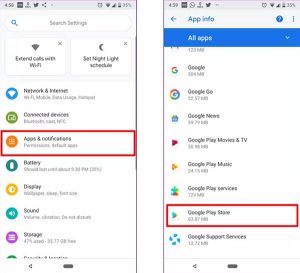The composite image consists of two side-by-side screenshots taken from an Android phone's settings interface. 

**Left Image:**
A red rectangular box highlights the 'Apps & notifications' section in the middle-left portion of this screenshot. This screen is part of the phone's settings menu, showcasing various settings options. From top to bottom, the listed settings include:
1. 'Network & internet' accompanied by a circular Wi-Fi symbol to the left.
2. 'Connected devices'
3. 'Apps & notifications'
4. 'Battery'
5. 'Display'
6. 'Sound'
7. 'Storage'

**Right Image:**
Similarly, a red rectangular box focuses on the words 'Google Play Store' in this screenshot. This screen seems to display information about various apps installed on the device. At the top center, the word 'Google' is visible, followed by a list of Google apps:
1. 'Google'
2. 'Google Go'
3. 'Google News'
4. 'Google Play Movies & TV'
5. 'Google Play Music'
6. 'Google Play Services'
7. 'Google Play Store' (highlighted)
8. 'Google Support Services'

In the upper-right corner, the term 'App info' is written in blue, below which is a label 'All apps' in white on a blue background.